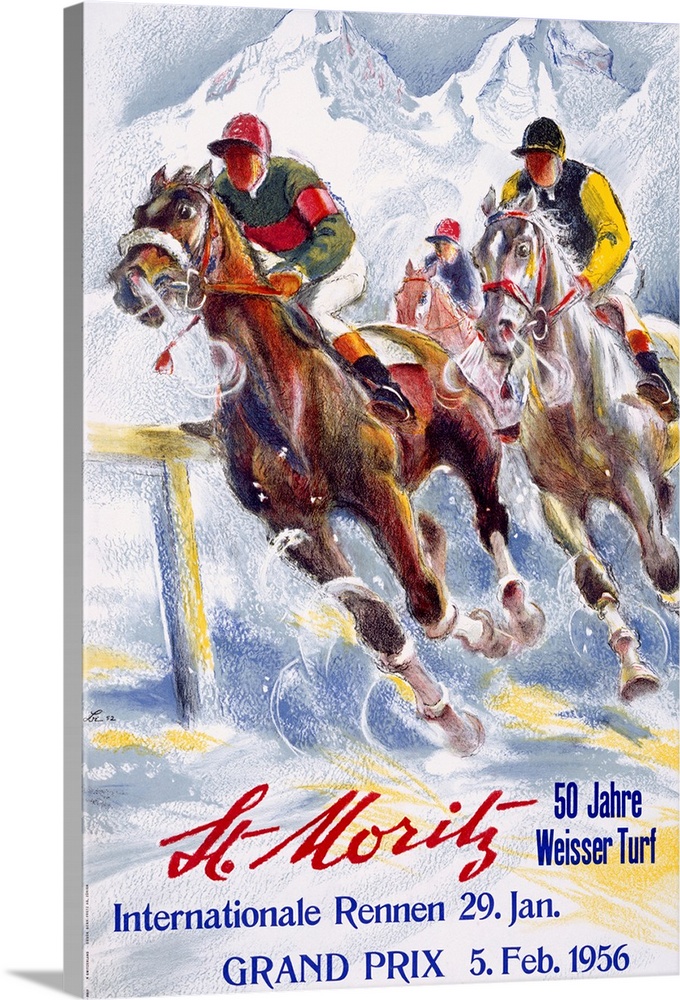The image is a detailed painting that resembles a book cover or poster with vivid dimensions. It captures an intense horse race set against the stunning backdrop of ice-capped mountains, suggesting a location in the Swiss Alps. 

Three jockeys are in the midst of the race on a snowy track. The lead jockey, riding a brown horse, is dressed in a red and green striped shirt, red hat, white pants, and gold and black boots. Following closely behind is a jockey on a white horse, clad in a black vest, yellow sleeves, and white pants. The third jockey, further back, is on a lighter brown horse and wears a blue jacket with a red hat. 

The text at the bottom of the image reads "St. Moritz Internationale Rennen" with additional details indicating that it’s an advertisement for an event that took place on the 5th of January, 1956, with the words "Grand Prix" prominently displayed.